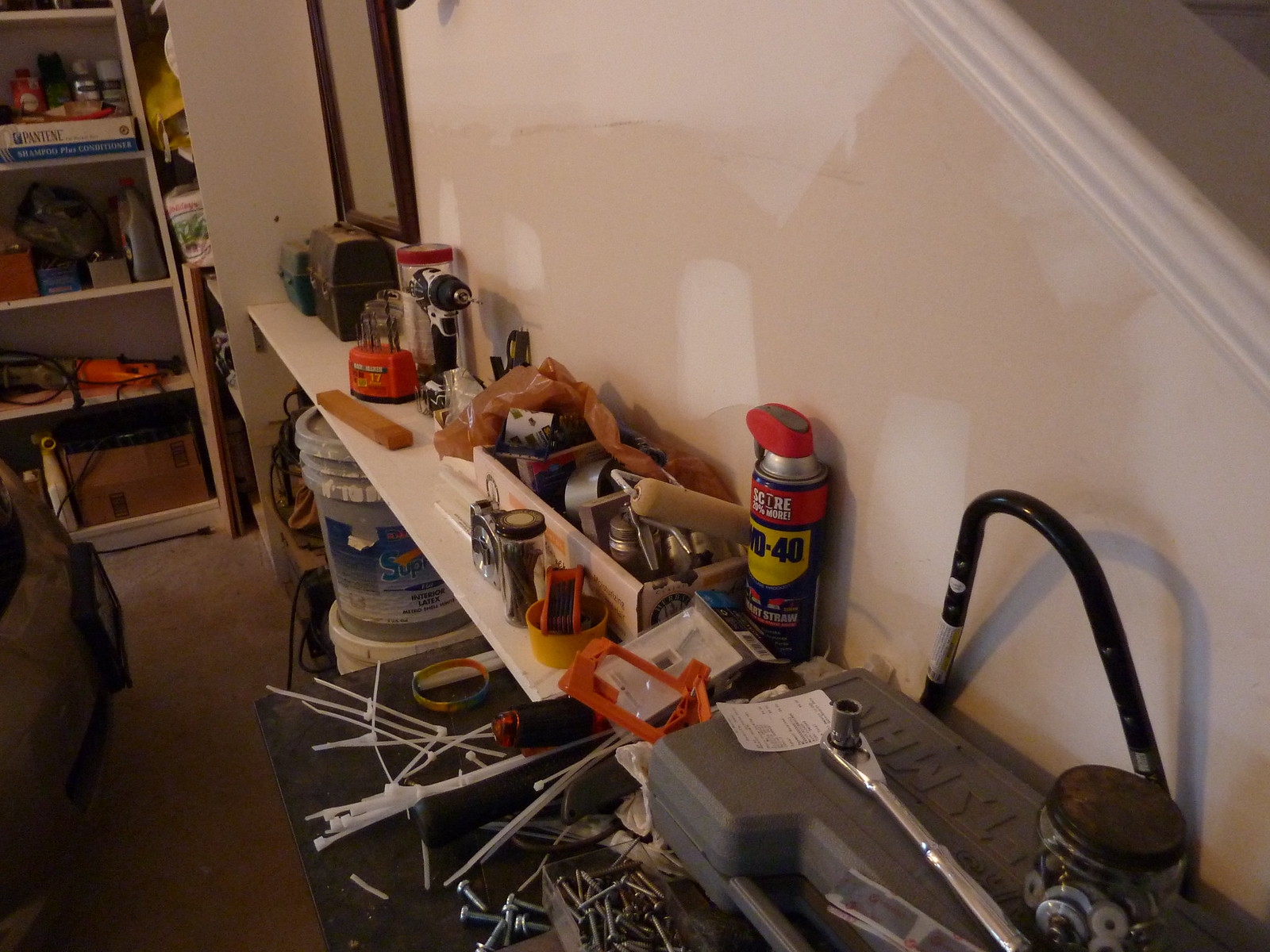In this high-resolution image, we are given a detailed view of a meticulously organized garage workspace. On the left-hand side of the frame, the front end of a car is visible, indicating that the garage also serves as a vehicle storage area. Mounted on the left wall is a white bookcase, stocked with an assortment of bottles that appear to be automotive fluids or household cleaning supplies. 

Adjacent to the right wall, there is a long white table that showcases an impressive array of drills and toolboxes, neatly lined up, ready for use. Among these tools, a can of WD-40 is prominently visible, alongside a paint roller and a jar filled with nails.

Nearer to the camera, there is a larger gray table that holds a collection of items including a pile of zip ties, various screws, and another toolbox. Positioned closest to the camera on the right is a jar brimming with washers, demonstrating a well-equipped and orderly workspace, ready for any project that might come its way.